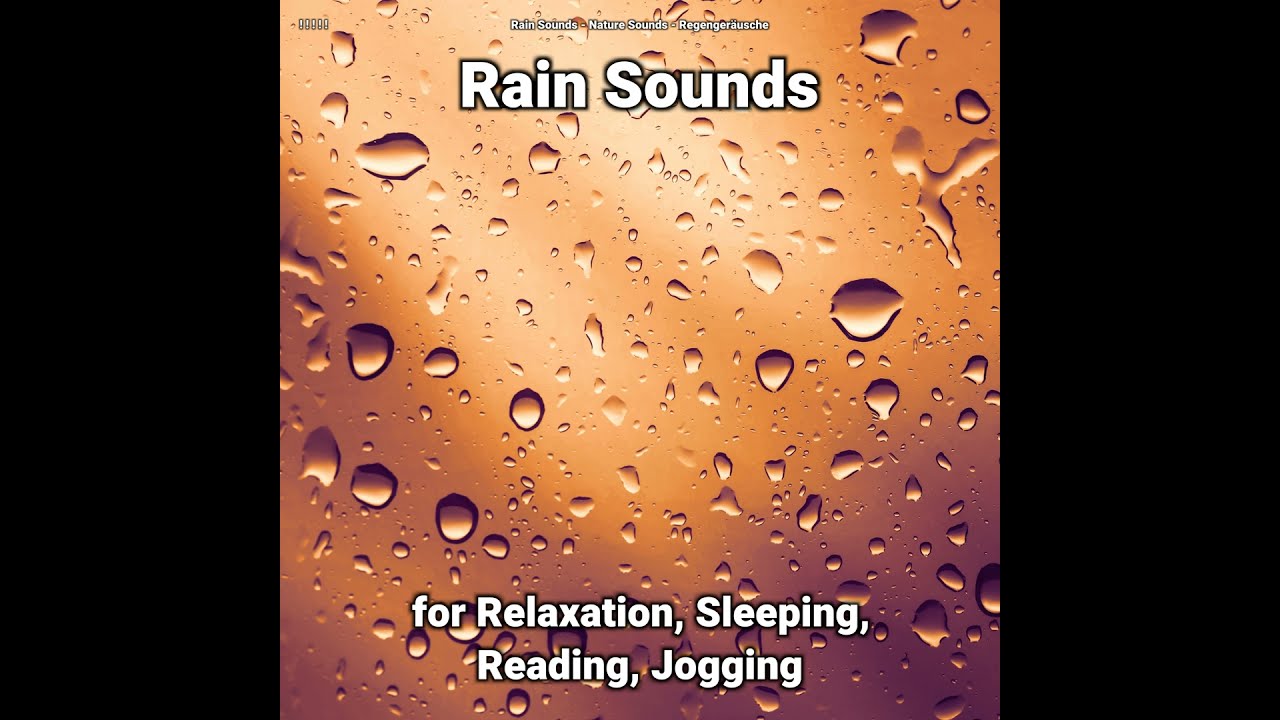The image depicts a calming advertisement for a rain and nature sounds app. The central focus is a photograph of rain-splattered droplets on what appears to be a camera or window lens. The background features a diffused blend of purplish and peachy hues, with translucent raindrops of various sizes scattered throughout, appearing both in large and small forms. The sides of the image are bordered by vertical black bars that take up about a fourth of the photo each. 

At the very top of the image, there is small white text that reads "rain sounds, nature sounds." Beneath this, in larger, bolder white letters with a black border, it prominently says "RAIN SOUNDS." At the very bottom, more white text with black borders states the app's intended uses: "FOR RELAXATION, SLEEPING, READING, JOGGING," with the initial letters of these words capitalized. The entire composition exudes a tranquil and serene atmosphere, emphasized by the soft, muted colors and the gentle depiction of raindrops.